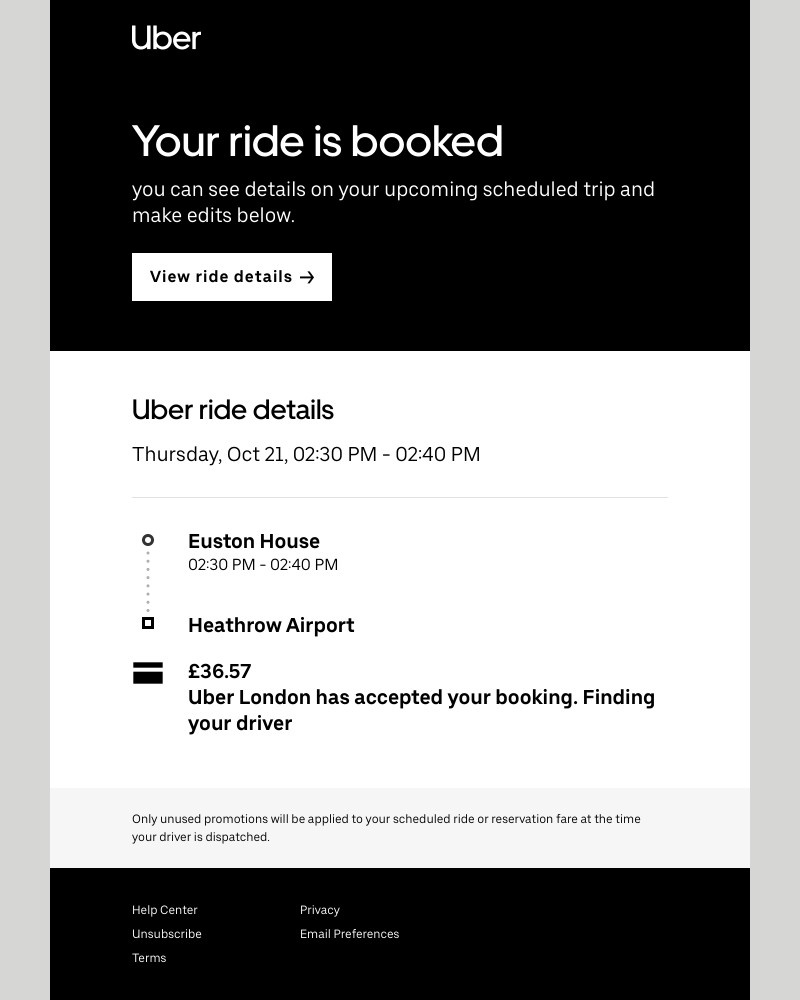This is a descriptive and detailed caption for the image:

---

This image is a screenshot of an Uber confirmation page. At the top, there is a sleek black banner with the Uber logo in white lettering. The text reads, "Uber, your ride is booked." Just below, there's a message stating, "You can see details on your upcoming scheduled trip and make edits below." Below this message is a prominent white button labeled "View Ride Details."

Further down, the screen displays specific details about the scheduled Uber ride. The trip is set for Thursday, October 21st, with a pick-up time frame between 2:30 PM and 2:40 PM. The journey is from Euston House to Heathrow Airport. The total fare for this ride is £36.57. It also notes that Uber London has accepted the booking and is in the process of finding a driver.

Additional information mentions that only unused promotions will be applied to the scheduled ride or reservation fare at the time the driver is dispatched. 

At the bottom of the confirmation page, there are several links including "Help Center," "Unsubscribe," "Terms," "Privacy," and "E-mail Preferences."

In summary, this structured and detailed booking page ensures the passenger is well informed about their upcoming journey, fare, and various options to modify or seek assistance regarding their trip.